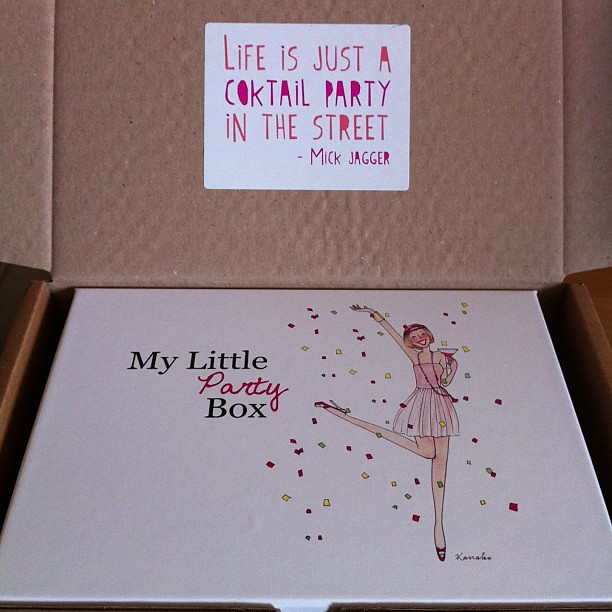This image depicts a white box with a festive design. The lid features a white background adorned with a colorful illustration of a girl in a pink, short party dress and high heels, holding a martini glass. Sprinkles of red, green, and yellow confetti surround her. Above the girl, there's a prominent sign in pink lettering that reads, "Life is just a cocktail party in the street." This quote is attributed to Mick Jagger, written underneath the phrase. The box itself, which is white, bears the title "My Little Party Box" with the word "party" highlighted in red cursive lettering. The confetti motif continues on the box's surface, enhancing the celebratory theme. The open lid reveals another plain cardboard box nestled inside.